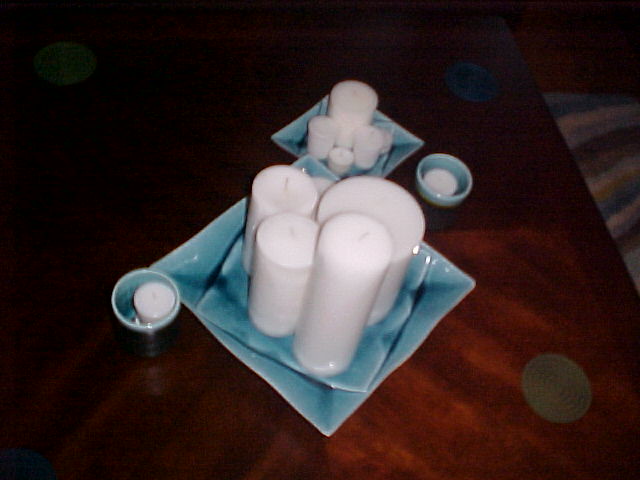The photograph showcases a richly hued mahogany table adorned with an array of candles set in elegant blue ceramic dishes. To the right of the table, a towel with bold yellow, white, and blue stripes adds a splash of color. On the table, there are two round blue containers, each holding a teacup candle. Centrally positioned towards the back is a square light blue porcelain tray that holds a large candle flanked by two medium candles and a teacup candle. In front of this, a larger light blue ceramic plate is nested with a smaller square plate in a pattern that creates a dish-within-a-dish appearance, both adorned with five white candles of varying lengths, ranging from one to five inches tall. Off to the side, a circular grey coaster and a grey and blue lined carpet further enhance the composition, contributing to the sophisticated and serene ambiance of the scene.